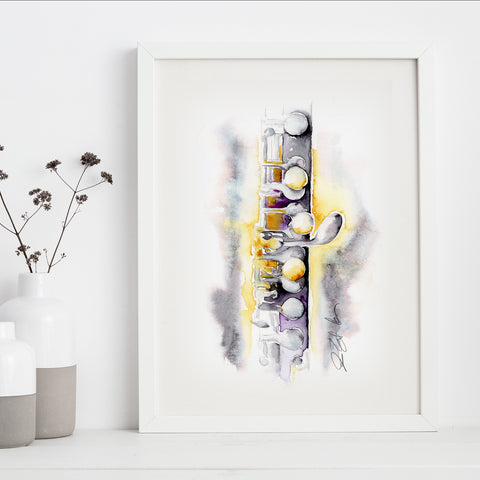In this minimalistic image, a photograph captures a serene setup on a creamy white background, all set on a white shelf. To the left, there are two cylindrical vases with white ceramic tops and gray terracotta bottoms. The larger vase, reaching from the bottom left corner towards the center, contains two delicate, dark brown flower stems. Adjacent to these vases, and slightly to the right, is a framed watercolor painting of a clarinet. The clarinet's detailed depiction includes predominantly silvery tones with subtle hints of yellowish-gold along the button parts, enhanced by shadowing in yellow and gray, giving it depth and dimension. The painting, bordered with a white mat and frame, features the artist’s signed initials in script to the left of the clarinet.